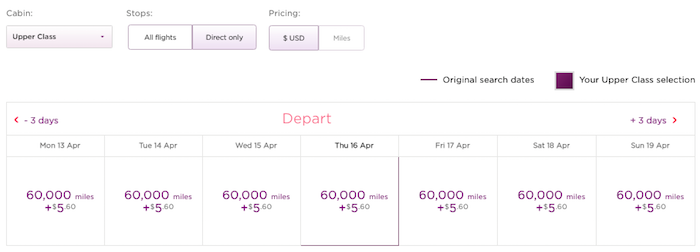This image appears to be a screenshot from a flight booking website. In the top left corner, there is a navigational bar containing three sections: "Cabin," "Stops," and "Pricing." Under each section, there are drop-down menus and options. 

1. "Cabin" features a drop-down menu displaying "Upper Class."
2. "Stops" offers two choices: "All Flights" and "Direct Only." The "Direct Only" option is highlighted.
3. "Pricing" includes buttons for "USD" and "Miles," with the "USD" button highlighted. 

Below this menu area, aligned to the right, there is a section labeled "Original Search Date" followed by "Search Dates." Adjacent to this is a purple square next to the text "Your Upper Class Selection."

The central part of the image displays a grid for selecting flight dates and corresponding details. On the left is a red arrow pointing to the left with a label "Minus 3 Days." The center prominently reads "Depart" in red text, and on the right is another red arrow pointing to the right labeled "Plus 3 Days."

Beneath this grid section, there are seven rectangles each representing consecutive dates: Monday, April 13th; Tuesday, April 14th; Wednesday, April 15th; Thursday, April 16th; Friday, April 17th; Saturday, April 18th; and Sunday, April 19th. Below each date rectangle, there are seven squares that display the pricing in a "Miles plus Money" format. For all listed dates, the cost is consistently indicated as "6,000 miles plus $5.60."

The overall layout suggests an interface for selecting and confirming flight availability and preferences, with specific emphasis on an upper-class flight option and direct flights priced in both miles and USD.